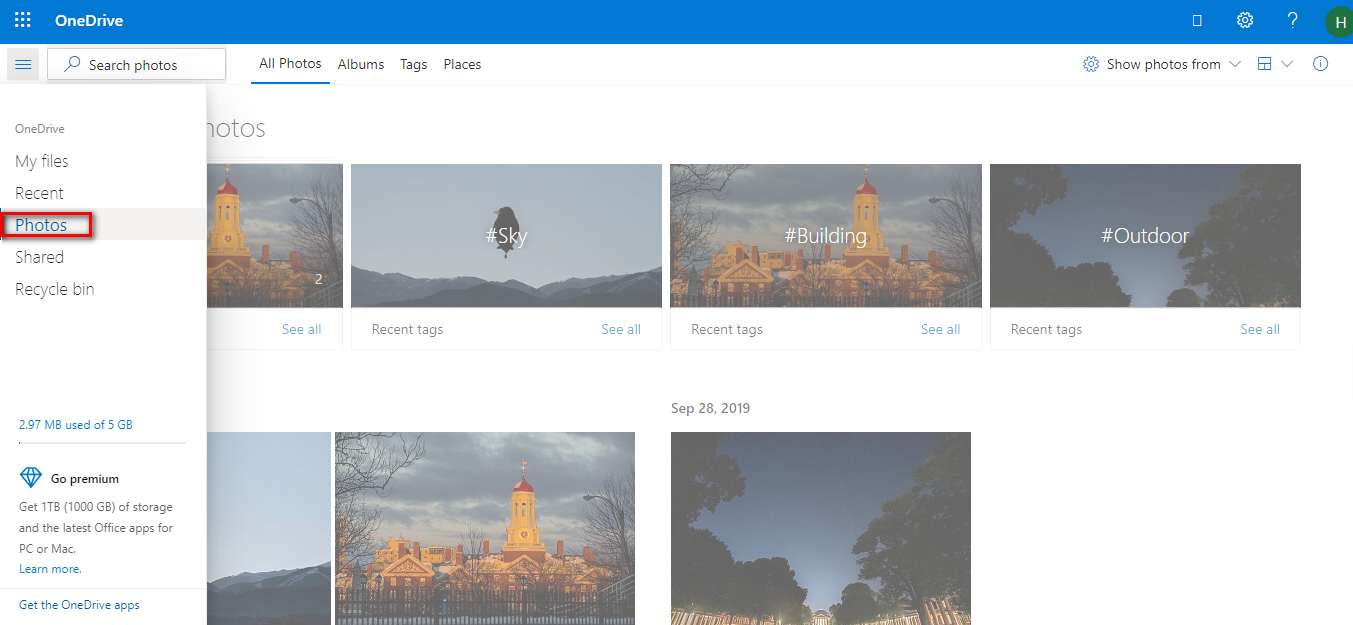The image appears to be a screenshot taken from a computer screen, showcasing a collage of multiple photographs arranged in a grid format. Dominating the background of many of these images is a distinctive town scene featuring a tall building, resembling a lighthouse, that rises above the other structures. This particular scene is evident in three of the photos—two positioned in the top row and one in the bottom row.

Additionally, there are two photographs titled "sky," each positioned diagonally from one another. These images portray a silhouette of land beneath a vast open sky. Alongside these, there are two more photos displaying the sky viewed through the trees. The images are differentiated by the presence of hashtags; one photo with the sky silhouette lacks a hashtag at the bottom, while the others include hashtags such as "#outdoor" at the top. Therefore, the duplicate instances of these pictures indicate one version with hashtags and added elements, while the other versions remain the original, unaltered images.